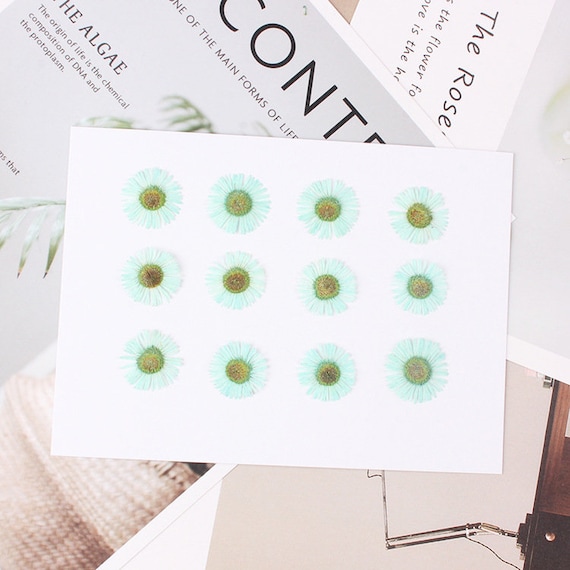The image is a visually intricate, vertically rectangular photograph with no definitive border or background. At the upper right corner, a business-card-sized piece of white paper is visible. Dominating the center is another piece of paper with a gray background and white trim, containing partially visible text that includes "C-O-N-T" and a reference to "the algae." The lower right corner features an indeterminate brown object with metal wire protruding from it. Central to the composition is a horizontally rectangular white piece of paper decorated with 12 daisies arranged in three rows of four. These daisies, with white and mint-green petals surrounding yellowish-green centers, create a striking focal point. Additional text fragments, such as "the rose" and "the origin of life is the chemical composition of DNA and the protoplasm," appear on the paper, contributing to the complex and layered visual narrative of the image.